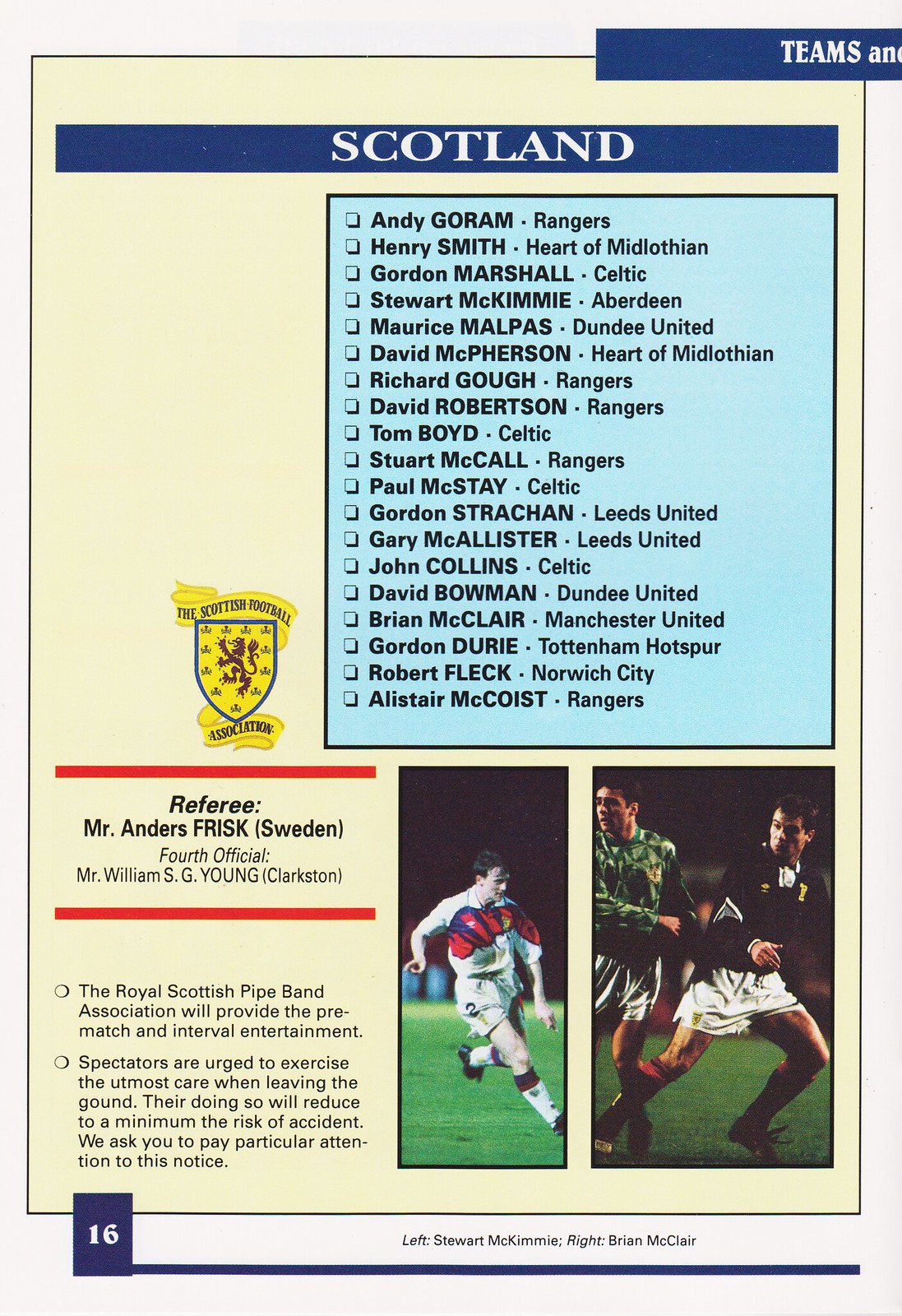The image is a detailed page from a magazine or pamphlet, displaying an off-white background with a page number '16' in a white font within a vertical blue rectangle on the bottom left corner. Dominating the middle of the page is a beige box with a vertical blue line at the top, where "SCOTLAND" is prominently displayed in white all-caps font. Below this, in a light blue background, is an extensive list of soccer players and their respective teams: Andy Gorham (Rangers), Henry Smith (Heart of Midlothian), Gordon Marshall (Celtic), Stuart McKimmy (Aberdeen), and many more. Noteworthy mentions include Maurice Malpast, David McPherson, Richard Gow, David Robertson, Tim Boyds, Stuart McCall, Paul McStay, Gordon Strachan, Gary McAllister, John Collins, David Baumann, Brian McClure, Gordon Ury, Robert Fleck, and Alistair McCoy. The list extends beyond the halfway point of the page. Below this, a section labeled "Referee" mentions Mr. Anders Frisk from Sweden and Fourth Official Mr. Williams SG Young Clarkson, accompanied by two smaller paragraphs of information. Additionally, there are two images of soccer players in action on the right side. A brief legend at the bottom identifies these images: "Left: Stuart McKimmy, Right: Brian McClure." This page resembles a well-organized informational section about Scottish soccer, combining player listings, referee details, and dynamic imagery.